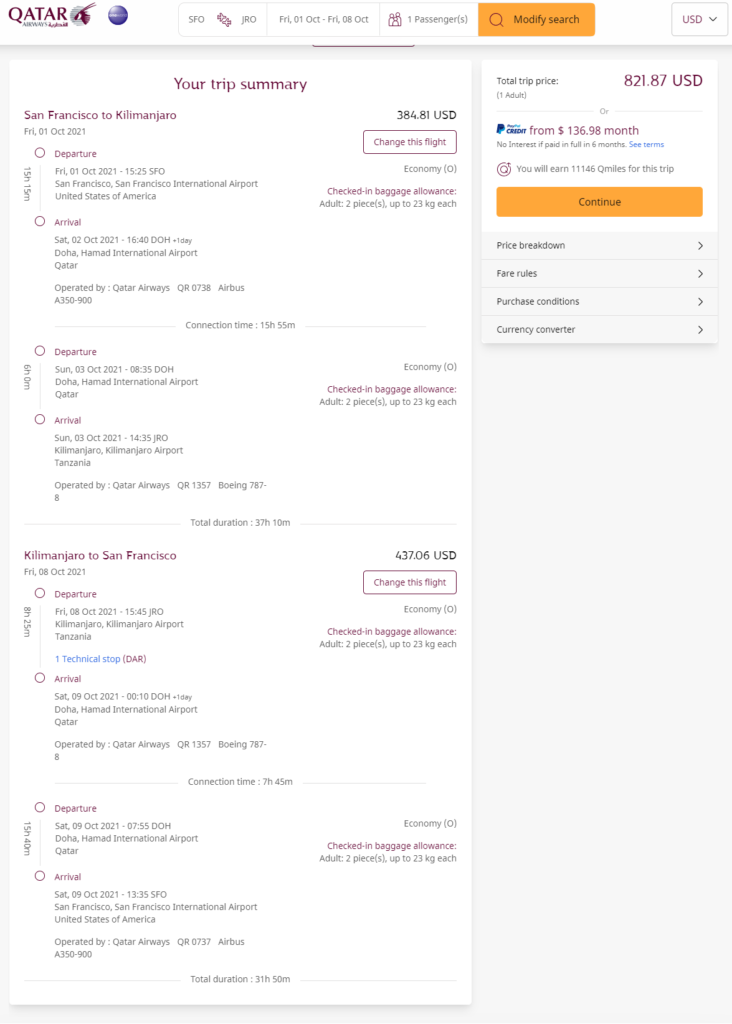The image displays a detailed trip summary on the Qatar Airways website for a passenger traveling from San Francisco to Kilimanjaro. The one-way flight is priced at $384 and includes specific details such as the departure date and time, arrival date and time, and information about a connecting flight with its respective departure and arrival times. The class of service is specified as Economy. 

The return leg of the journey from Kilimanjaro to San Francisco also lists the departure and arrival dates and times, along with details about a connecting flight. Under each flight segment, there are buttons available for modifying the flight arrangements.

The total cost of the round trip is indicated as $821, with an option to split the payment into monthly installments of $136. A prominent "Continue" button is present, allowing the user to proceed with finalizing the travel plans.